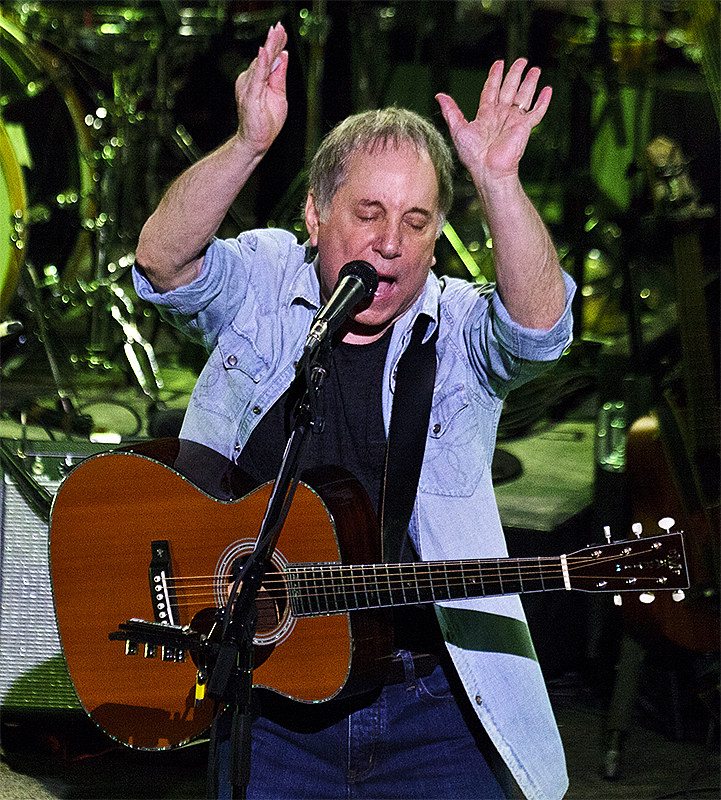The image captures a close-up of a man performing passionately at what appears to be a concert stage, although the background is blurred. His light brownish-blonde hair flows freely as he sings with his mouth wide open and eyes shut, fully immersed in the moment. The man is dressed in blue jeans paired with a blue denim jacket that is rolled up at the sleeves, underneath which he wears a black polo shirt. He stands dynamically, hands raised in the air—his right hand gripping a pick meant for strumming his wooden lead guitar, which hangs from a strap around his neck. The background, though indistinguishable, shows shades of green, making it ambiguous whether he is indoors or outdoors. Notable details include what seems to be a set of drums positioned at the top left of the image. The man’s attire and stance give a vibrant energy to the performance, evocative of an immersive musical experience.